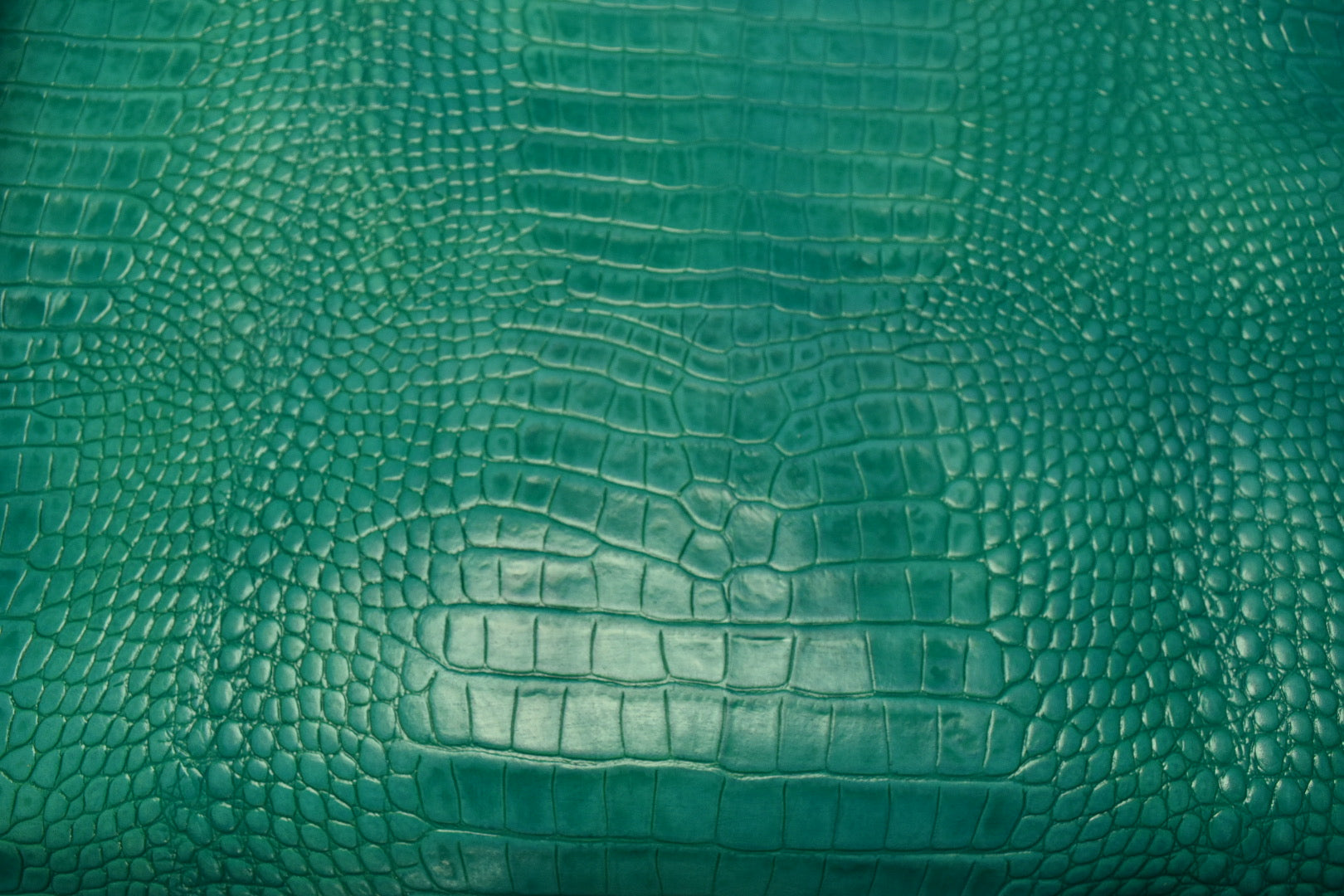The image is a horizontally rectangular close-up of what appears to be a treated reptile skin, possibly from an alligator, crafted into an object like a purse or bag. The skin is dyed a vibrant turquoise color, although some have also observed hints of a bright evergreen shade. The pattern of the scales varies across the image; in the center, the scales are larger and square-like, while towards the left and right edges, they become smaller and more circular, with some teardrop shapes interspersed. The scales all share the same basic color, with subtle shading variations. There is no distinctive border or background visible in the image, and artificial light slightly illuminates the bottom-left of the center, adding a reflective sheen to the texture.